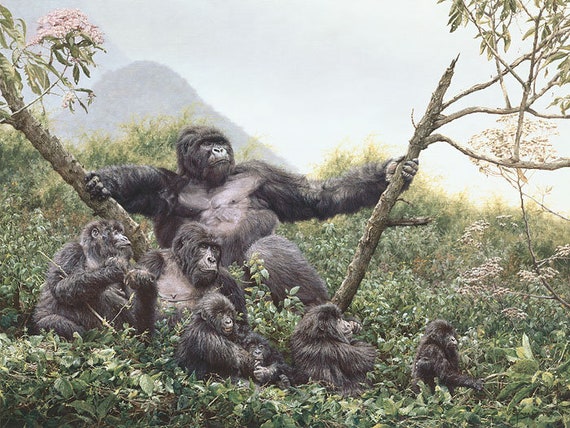A highly detailed illustration depicts a family of seven gorillas situated high in the treetops, surrounded by lush forest vegetation. At the center of the composition is a large male gorilla, prominently featured, leaning back and grasping two tree branches, seemingly bending them with his immense strength. His eyes are closed, as if in a moment of tranquility, while his family gathers around him. Below him, there are five smaller gorillas, including two medium-sized ones and three baby gorillas, all nestled among a wealth of green foliage, grasses, and leaves. A tree branch adorned with pink flowers adds a splash of color to the scene. In the distance, towering mountains stand under a sky tinged with hues of gray, green, yellow, pink, white, and orange, enhancing the landscape-like quality of the illustration. The overall atmosphere suggests a serene and cohesive family moment amidst the dense and vibrant forest canopy.